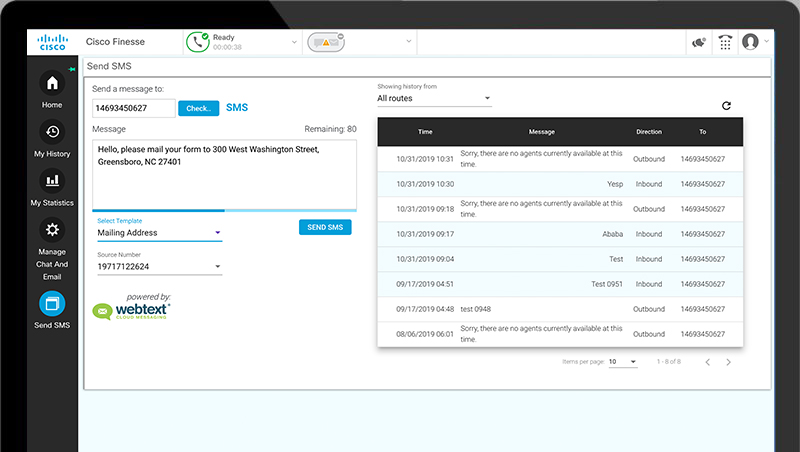The image is a rectangular interface screenshot, approximately 50% wider than it is tall, featuring a distinct black border. The central portion of the image depicts a windowed interface with a white background. In the upper left corner of this window, the Cisco logo is prominently displayed in light blue, characterized by its recognizable two-mountain bar design. Adjacent to the logo, the words "Cisco Finesse" are written in black text. 

To the right of the logo and text, there is a green circular phone icon with a green checkmark in its upper right corner, and the word "Ready" is printed beside it. Directly below this section is a timer showing "38 seconds."

On the left side of the interface, a black vertical navigation bar hosts several icons: a house symbol for the home page, a clock for viewing history, a bar graph for statistics, a gear for managing chat and email, and a box for sending SMS, the latter currently highlighted in blue.

The primary area of the screen, with a white background, is headed with a black title that reads "Send SMS." Beneath this title, in smaller text, it instructs users to "Send a Message to" followed by a blank field where a phone number is entered. To the right of this input field, a blue button labeled "Check" is available, and just beyond this button, "SMS" is displayed in blue text.